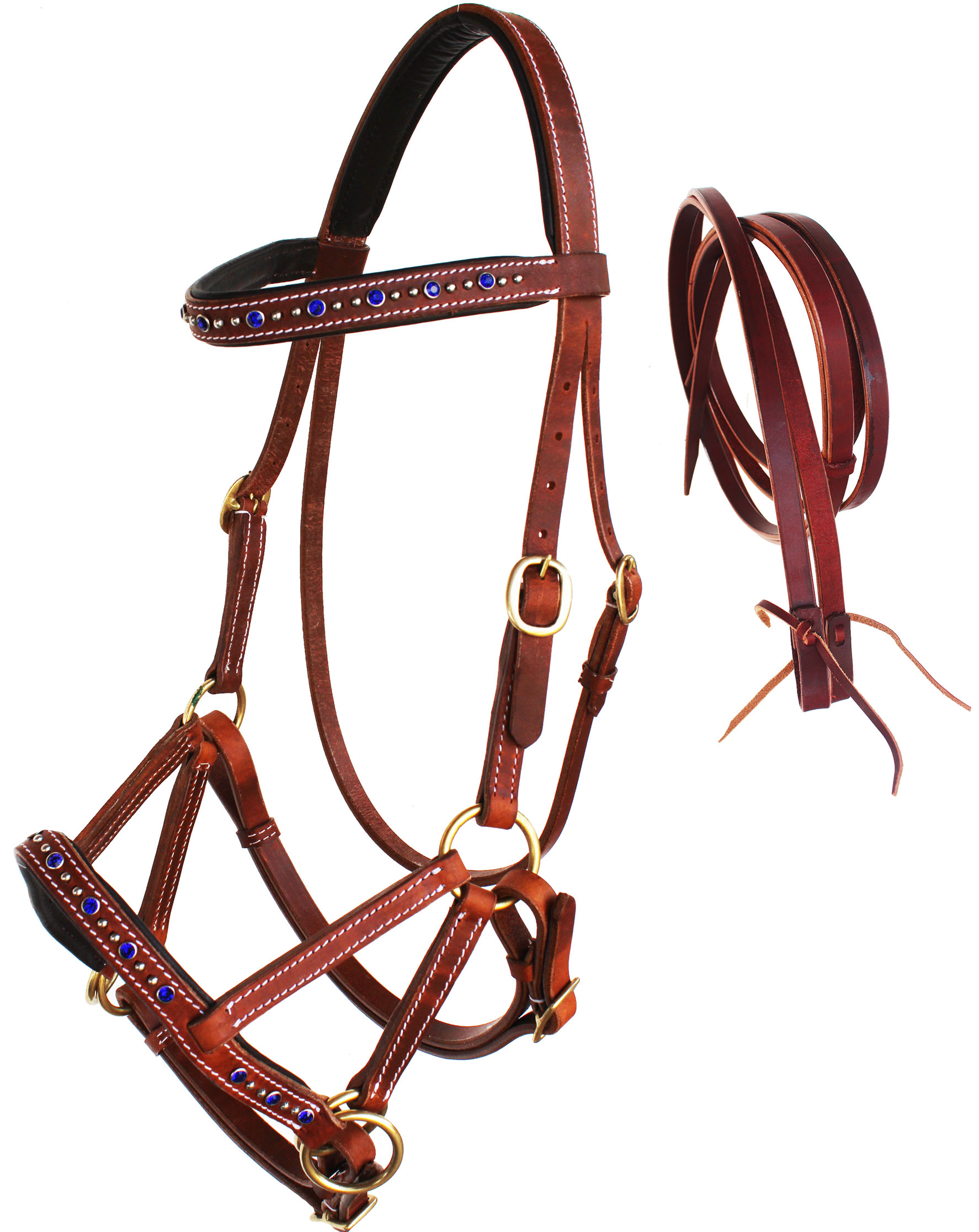The image is a realistic, studio-style photograph of a detailed leather harness set against a plain white background. This harness system is constructed primarily from dark brown leather and is intricately stitched with noticeable white thread. The harness features multiple brass or gold rings and buckles, which proficiently connect its parts together. It is adorned with blue gemstones and silver rivets in alternating patterns, adding a decorative touch to both the top and bottom sections of the harness. Off to the right of the main harness, there is an additional, coiled leather strap or belt that matches the dark brown color and detailing of the harness. The overall design, with its elaborate loops and ornamental blue jewels, suggests its possible use in horseback riding or could be a product for sale in a web advertisement, given its meticulously crafted appearance.